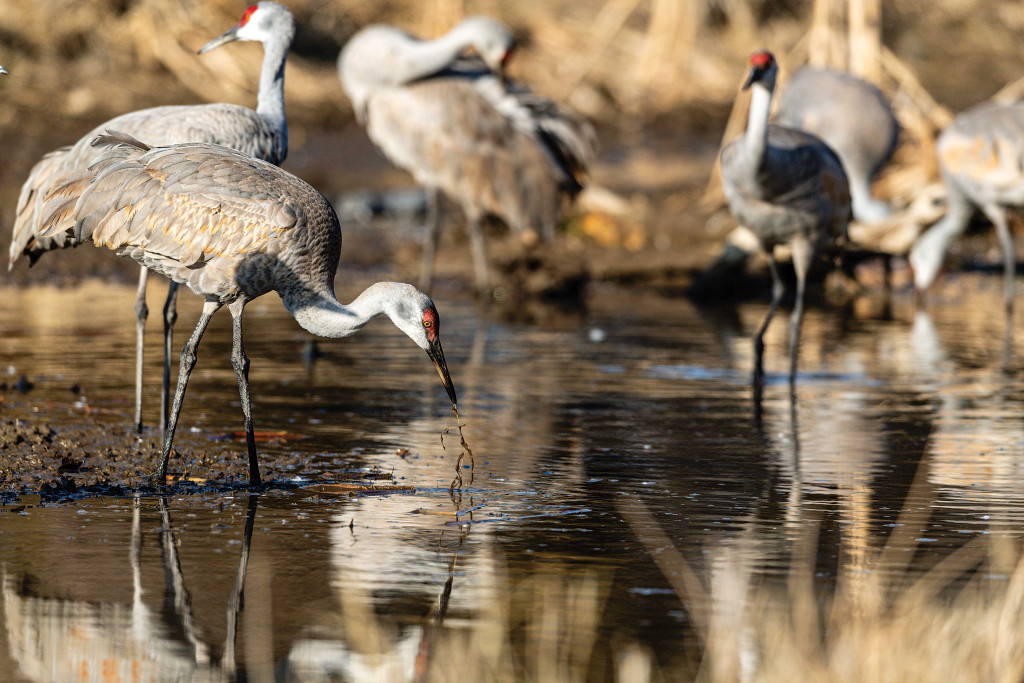In this image, we see a group of six water birds, resembling storks or cranes, wading through a shallow, dark-colored pond. These birds are characterized by their long, slender black legs and their distinctive plumage: white necks and heads, with bodies that are a blend of light brown, tan, gray, and hints of yellow. An orange spot is visible near the front of their heads, and they possess dark, long, pointy beaks and yellow eyes. One notable bird displays a red comb-like marking on its head, possibly identifying it as a male. Some of the birds stand upright, while others have their heads dipped into the water, seemingly searching for food. The scene is framed by straw-colored reeds and tall grasses both in the foreground and background, adding to the natural, somewhat marshy appearance. The water itself appears dark and murky, with brown dirt visible near the water’s edge, emphasizing the shallow depth of the pond.